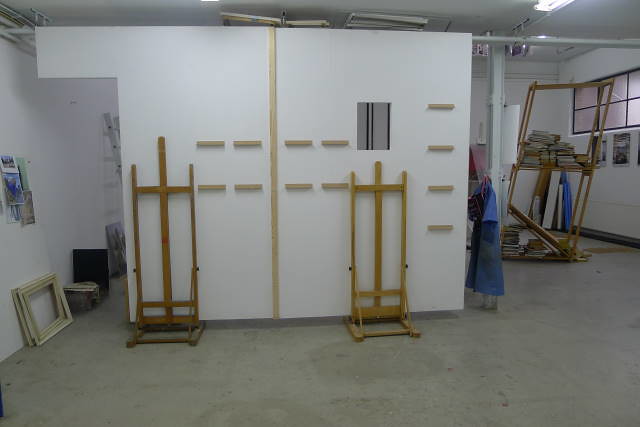The photograph captures a workshop or art studio with a concrete floor that’s a blend of dark gray and some marbled patches. The space is illuminated by white fluorescent lights on the ceiling. Against the white walls, there are several elements of interest. On the left side, there’s a collection of picture frames leaning against the wall, beneath some pictures tacked onto it. A piece of clothing, possibly a dress, hangs on a rack nearby.

In the focal area of the image, two wooden easels are set very low to the floor, holding a large, white rectangular canvas or partition with a small cut-out window on its right half. This canvas features little wooden notches across the middle and a wooden plank running down, suggesting it might be part of a set-building project. 

On the right side, against another white wall, there's a shelf filled with an assortment of items, leaning precariously towards a six-pane window trimmed in black. Below this window, additional pieces of artwork are placed, and the cluttered yet creative atmosphere is accentuated by the yellow wooden frames scattered around. Pipes run along the ceiling, contributing to the industrial feel of the space.